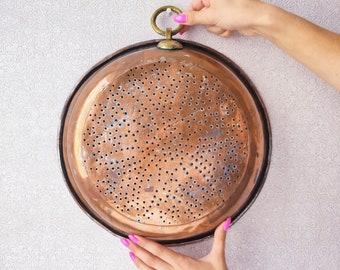This detailed photograph captures a woman's intricately manicured hands, with long, pink-painted fingernails, as she hangs a round, metallic object on a white wall. The object, which might be a vintage brass strainer or a decorative kitchen piece, features a distinctive flower pattern formed by punched holes on its darker-colored bottom. This floral design is crafted into the brass or copper, creating an artistic visual. The rim of the object is noticeably darker than the rest of its brass body, adding contrast. The woman’s right hand is carefully hooking the brass ring at the top of the object onto a white peg on the wall, while her left hand supports the object from below. The metallic sheen and the detailed flower design make this piece an eye-catching artifact against the plain white backdrop.